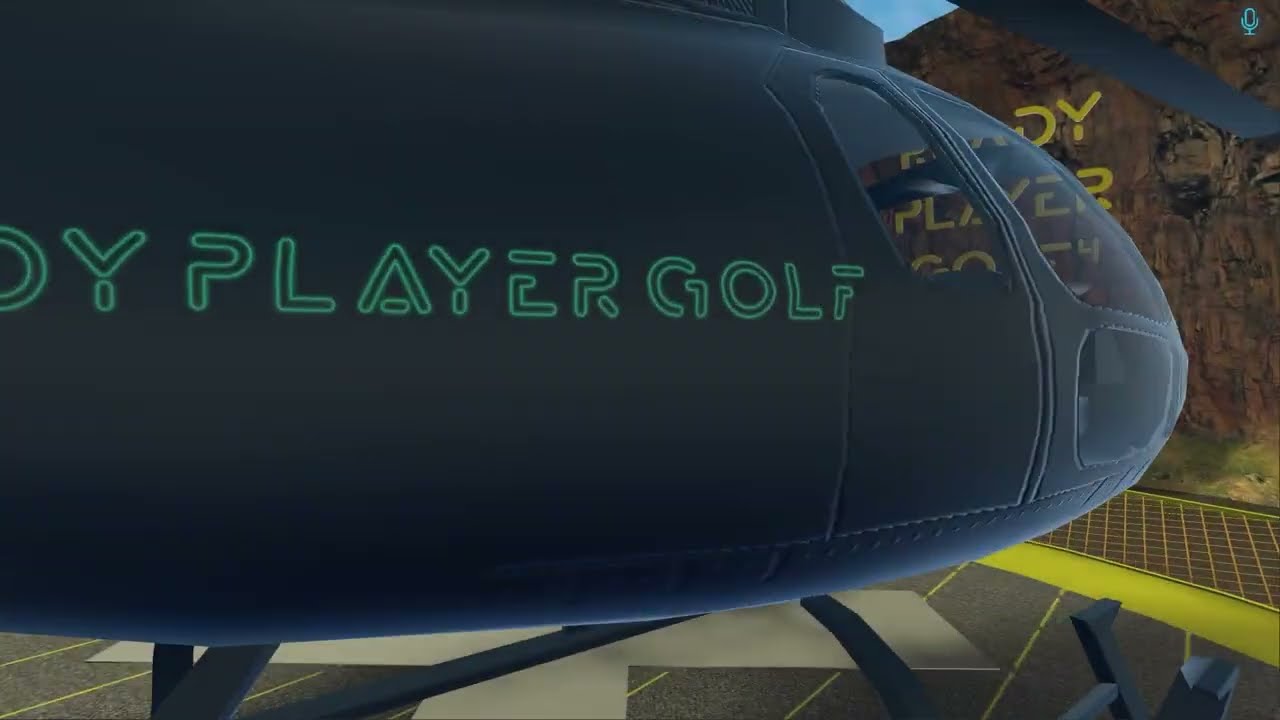The image depicts a close-up of a dark gray helicopter, likely computer-generated or from a video game, situated on a concrete slab marked with a white "X." The helicopter's side is prominent, with visible rivets and a portion of a rotor in the top right corner. In the background to the right, there's a rock cliff with yellow text partially obscured by the helicopter. This text, appearing in neon lights, reads "Ready Player Golf," although the first word is cut off, leaving "D-Y" visible. The words "player golf" are also inscribed across the helicopter itself, further enhancing the scene's digital or animated aesthetic. The rock cliff and helicopter's base are outlined with a yellow line, adding to the detailed composition of the image.